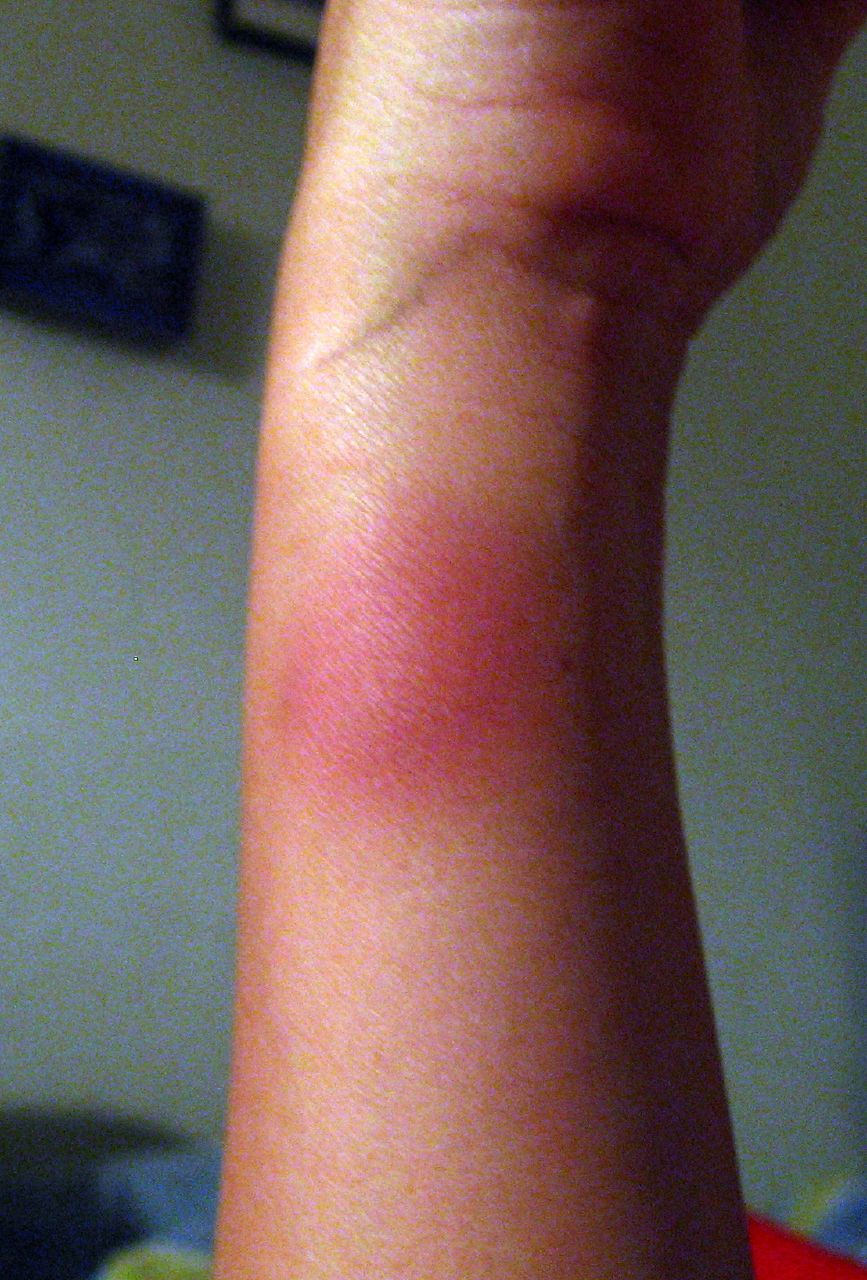The image is a close-up photograph of a light-skinned person's arm, taken from just below the elbow to just above the wrist, where the top of the hand is visible but no fingers are shown. The central focus is a large, swollen, and irritated bump on the arm, which is notably dark pink and appears painful. This bump could possibly be a bug bite, burn, or a rash. In the background, you can discern a white wall adorned with something black and blue, along with subtle hints of yellow and red, although these elements are not in focus. The overall quality of the picture is somewhat grainy and unprofessional, suggesting that it may have been taken quickly, perhaps to show a medical professional. The predominant colors in this image are the peach and pink tones of the person's skin and the inflamed bump.